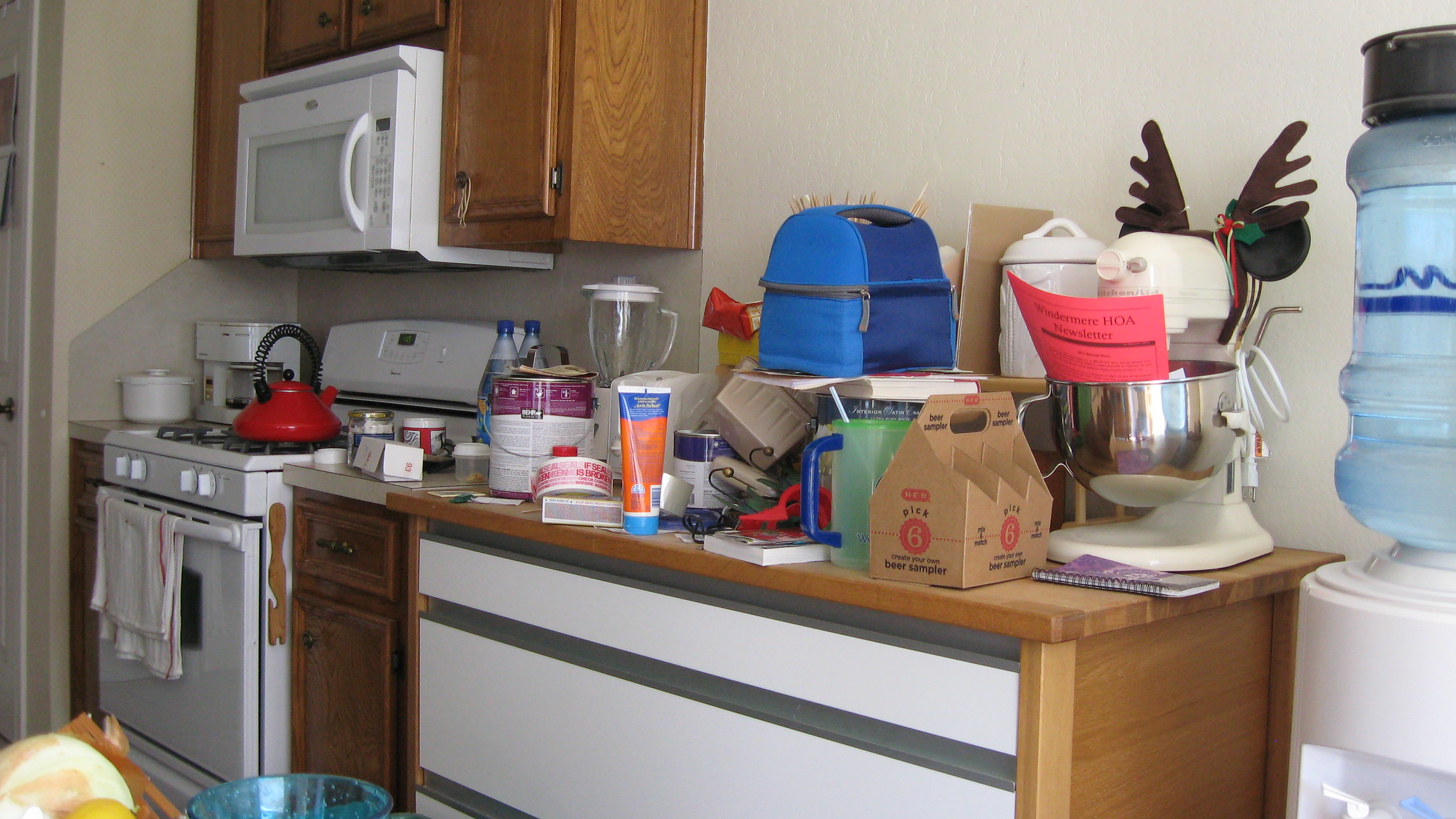This photograph showcases a kitchen in disarray, with various items scattered across the space. On the right side, a large water dispenser with a white base and buttons is visible. Adjacent to it is a brown wooden countertop with black and white lines at the front. Atop this counter, there is a white and silver mixer, a blue lunchbox, a cardboard box, several miscellaneous bottles, a can of paint, and a blender.

To the left of the countertop, a white stove with black accents stands out, featuring a red kettle on its surface and a towel hanging from its front. A small section of counter space next to the stove holds an unidentified white object. Above the stove, brown cabinets frame a white microwave. The kitchen walls are painted white, adding to the overall brightness of the room.

In the lower left corner of the photograph, various objects clutter the floor, including a clear blue item, and a mixture of white, yellow, and brown objects, contributing to the room's untidy appearance.